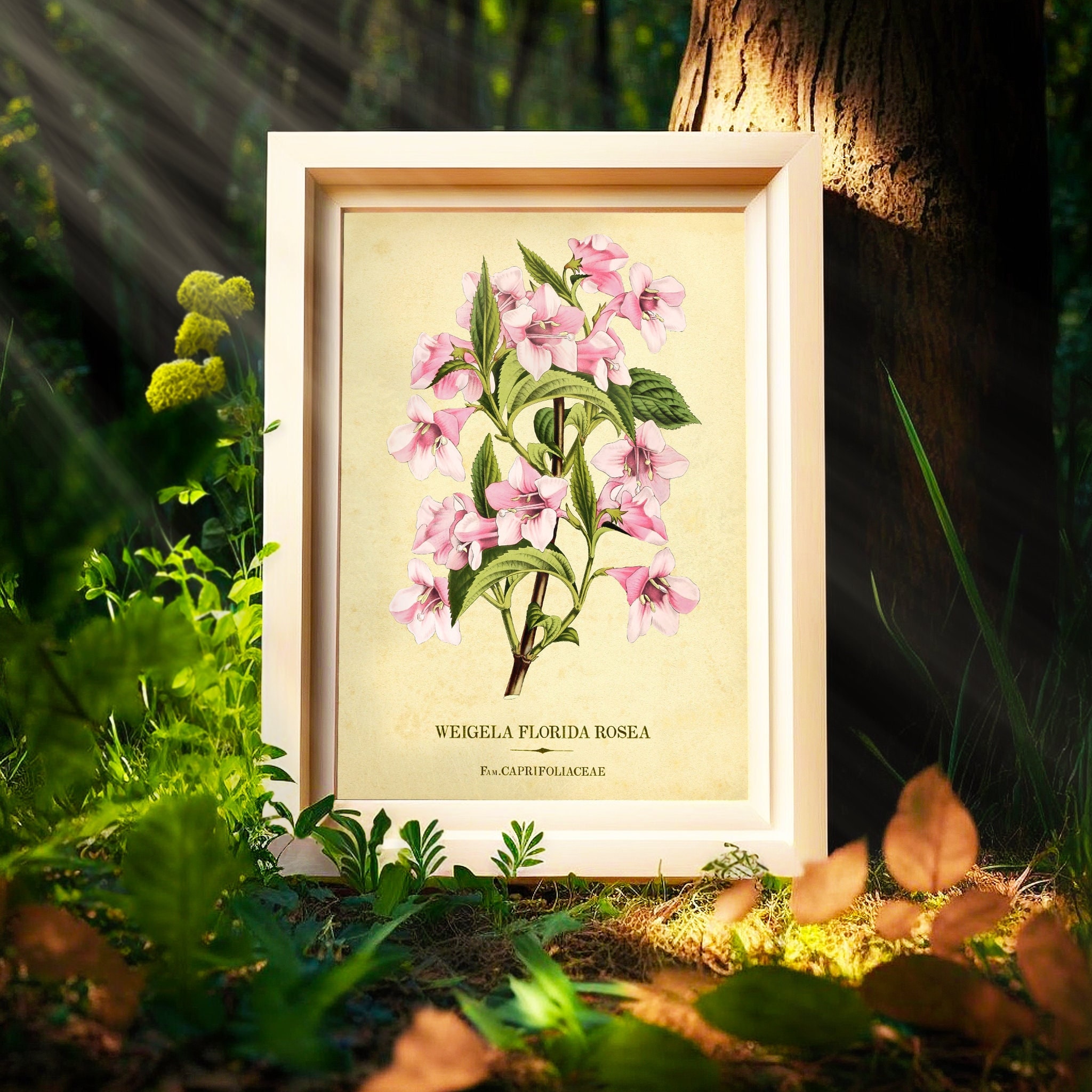This is an outdoor image of a meticulously framed and matted picture depicting the "Weigela florida rosea" plant, leaning against the base of a large tree trunk. The vibrant and vivid artwork showcases tall, thin stalks adorned with slim green leaves and clusters of trumpet-shaped flowers in shades of pink and purple. The frame, prominently detailed with multiple, stepped mats in a pinkish-white hue, enhances the delicate beauty of the floral subject. Set against the lush backdrop of a forest, the scene is bathed in sunlight streaming down from the left, illuminating the detailed print. Around the frame, patches of moss and small greeneries intermingle with scattered brown leaves, contributing to the natural and serene ambiance. The background fades into the darker greens and browns of the forest, encapsulating the framed picture and accentuating its botanical elegance.